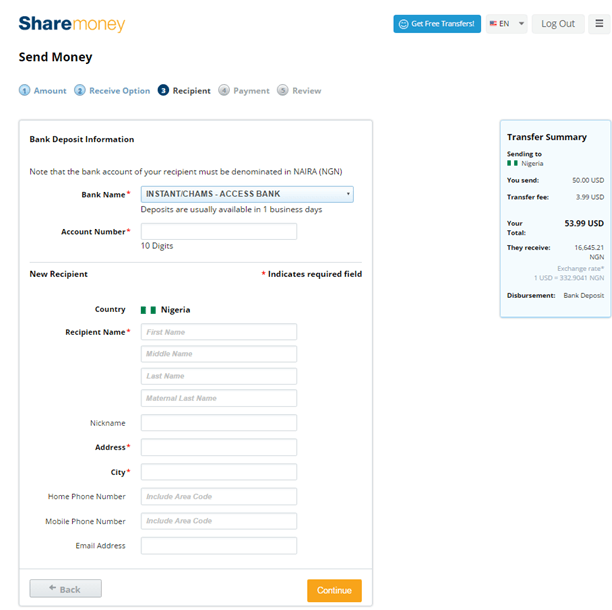The webpage titled "Share Money" features a sleek and organized interface with clear navigation options. At the header, "Share" is highlighted in blue, while "Money" is showcased in a gold-yellow hue. Positioned to the right is a prominent blue button with white text reading "Get Free Transfers." Next to it, there's a dropdown menu for selecting languages, defaulting to English, alongside a "Logout" link and a context menu.

Beneath the "Share Money" banner, users can access the "Send Money" section, featuring input fields such as "Amount" and "Receive Options," both highlighted in blue. The "Recipients" section displays a dark blue circle with a white numeral "3." Two buttons, "Payment" and "Review," are grayed out, indicating their current inaccessibility.

The "Bank Deposit Information" section specifies "Instant Chams Access Bank" as the bank name, awaiting a 10-digit account number. Required fields are marked with red asterisks. The recipient details include fields for "Country" set to Nigeria, potentially suggesting a notorious scam involving a so-called Nigerian Prince. The form collects "First Name," "Middle Name," "Last Name," "Maternal Last Name," "Nickname," "Address," "City," "Home Phone Number," "Mobile Phone Number," and "Email Address."

At the bottom, a grayed-out "Back" button and an orange "Continue" button (with white text) are positioned on the lower right. To the right side, a summary of the transfer is displayed, detailing that sending $50.00 with a $3.99 transfer fee totals $53.99. The recipient will receive ₦16,645.21, based on an exchange rate of 1 USD to 332 NGN, with disbursement through a bank deposit.

Overall, the webpage presents a comprehensive and user-friendly layout, clearly outlining the steps and details involved in sending money internationally.